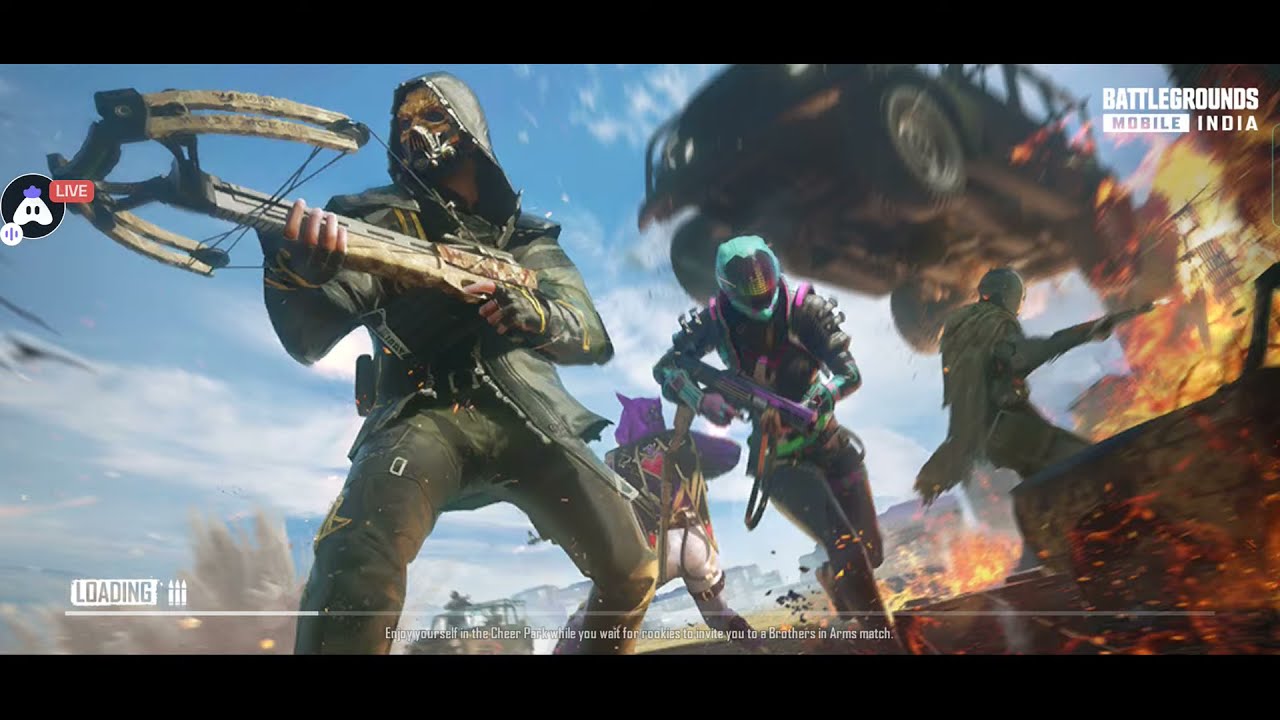The image is a detailed screenshot from the video game "Battlegrounds Mobile India," with the game title in all caps at the upper right corner. A black band across the top and bottom adjusts the vertical dimensions, giving it a widescreen look. At the bottom of the image, a loading bar is visible, about a quarter full, foreshadowing the game's imminent start. The text near the bar reads, "enjoy yourself in the cheer park while you wait for rookies to invite you to a brothers in arms match."

The main action centers around heavily armed characters in dynamic poses. Front and center is a character in dark green jacket and pants, wielding a crossbow-like weapon. He has a hood over his head, a gas mask covering his face, and penetrating dark eyes on tan skin. Behind him are three more characters in diverse combat gear: one with black body armor accented with teal and purple, a teal full-face shield helmet, and a purple gun; another character in white pants, a black vest, and a purple hoodie facing away; and a silhouetted figure in a raggedy jacket and dark pants, seemingly jumping with arms raised.

High above this chaotic scene, a large black Jeep is soaring through the sky, appearing to have launched off a cliff. Flames and explosions light up the right side of the image, adding to the sense of intense action, while the sky in the background is a mix of blue and white clouds. On the lower right, a wrecked car further emphasizes the war-torn environment.